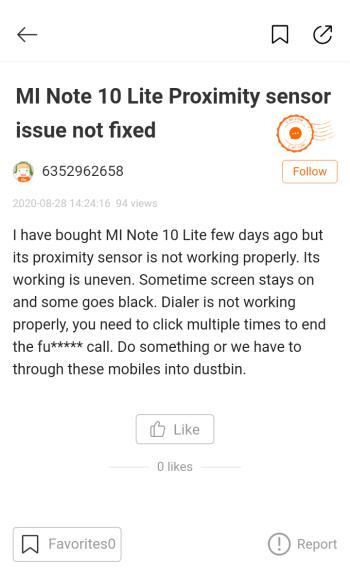Screenshot from a Website Highlighting an Issue with M.I. Note 10

At the top of the screenshot, there's an arrow pointing to the left. Next, there appears to be a flag-like icon, followed by a circular icon with an upward-pointing arrow, indicating the number 2 in the manner of a clock. A horizontal line separates these elements from the rest of the content. The background is predominantly white.

The central text prominently reads: "M.I. Note 10, White Proximity Sensor Issue Not Fixed." In this title, the "M" and "I" in "M.I." are capitalized, the "N" and "O" in "Note" are capitalized, the number "10" is depicted numerically, and both "L" in "Light" and "P" in "Proximity" are also capitalized.

Beneath the title, there is a small user icon followed by a numeric identifier: "635-296-2658." On the opposite side, the word "Follow" is displayed in orange text. Below this, the user has posted a detailed complaint:

"I have bought M.I. Note 10 a few days ago, but this proximity sensor is not working properly. It’s working is uneven. Sometimes screen stays on and some goes black. Dialer is not working properly. You need to click multiple times to end the F***ing call. Do something or we have to throw these mobiles into dustbin."

At the bottom of the screenshot, options to "Like," "Favorite," and "Report" the post are provided.